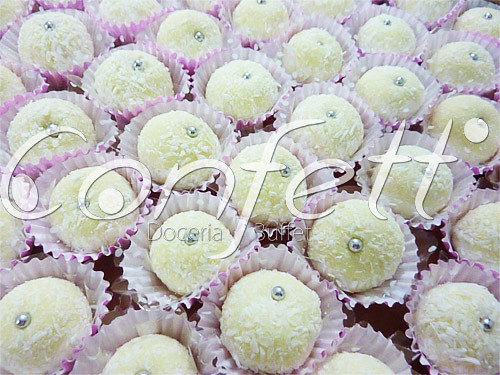The photograph captures a vibrant display of identical pastries arranged on a dark brown surface. Each pastry is a round, yellowish ball adorned with white flakes, and at the center of every pastry sits a single silver ball. These delectable treats are nestled in purple, ridged paper cupcake cups, adding a touch of color to the presentation. Superimposed on the image in elegant white cursive font is the word "confetti," with "Docheria Buffet" in smaller fonts underneath, both serving as a watermark. The entire frame is devoted to these pastries, suggesting they are likely showcased from a sweet shop or confectionery.